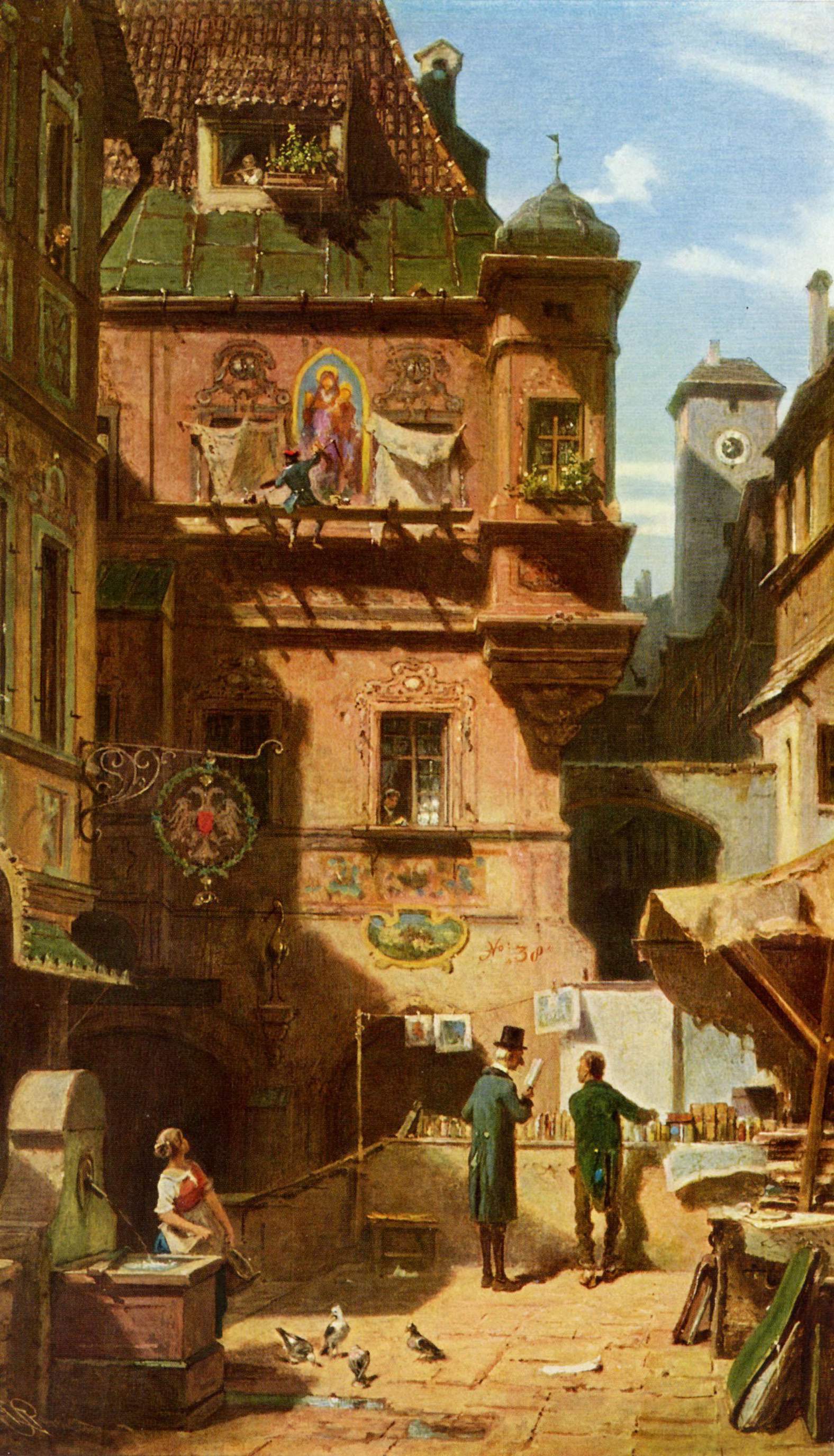This painting depicts a bright and vividly rendered courtyard scene, evocative of Dickens-era England or perhaps 19th-century Italy. The sky in the upper right-hand corner is a clear, bright blue, contrasting with the warm, terra cotta hues of the surrounding buildings. The courtyard is bustling with life, characterized by a sense of light and shadow interplay. 

In the lower part of the courtyard, two men are engaged in conversation; one is notably wearing a top hat and a green jacket. At their feet, pigeons peck at the ground. Nearby, a peasant gazes upward, adding to the scene’s dynamic atmosphere. Further to the left, a woman is positioned by a fountain, looking up at a child who stands on a balcony above her.

The architectural details are intricate: the buildings are adorned in an orange-brown plaster, with distinct green accents. On the top story of one building, a figure peers out of a window surrounded by leafy plants. Below, an artist, identifiable by his blue outfit and red cap, is depicted painting an image framed in blue, believed to be of Christ.

The courtyard features multiple arched entryways and has a terra cotta texture that enhances its historical and atmospheric feel, reminiscent of a scene from a Dickens novel or a Roman novel from the 1840s. The painting’s detailed portrayal of daily life in this small courtyard is both engaging and rich in historical ambiance.